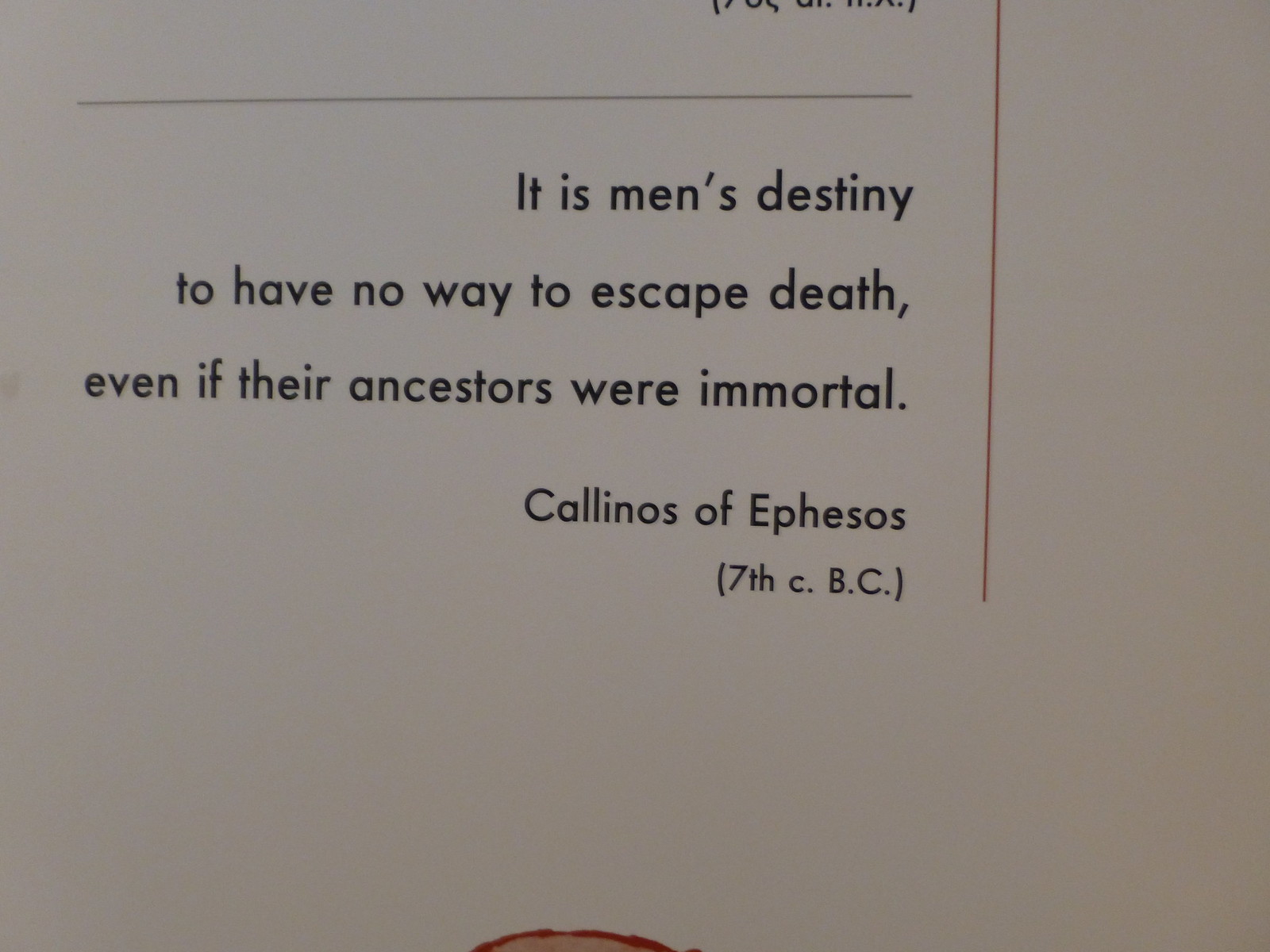The image is a close-up photograph of a partially visible piece of paper or sign displaying a quotation from a historical figure named Callinos of Ephesos, from the 7th century B.C. The text on the paper, right-justified and broken into three lines, reads: "It is men's destiny to have no way to escape death, even if their ancestors were immortal." Above the quote, a thin black horizontal line spans about two-thirds of the width of the paper, and a vertical red line borders the quote on the right, extending off the visible edge of the image. At the bottom, a yellow shape with a red outline is partially cut off. Additionally, the top center of the image appears to have more words that are also cut off by the photograph's edge.